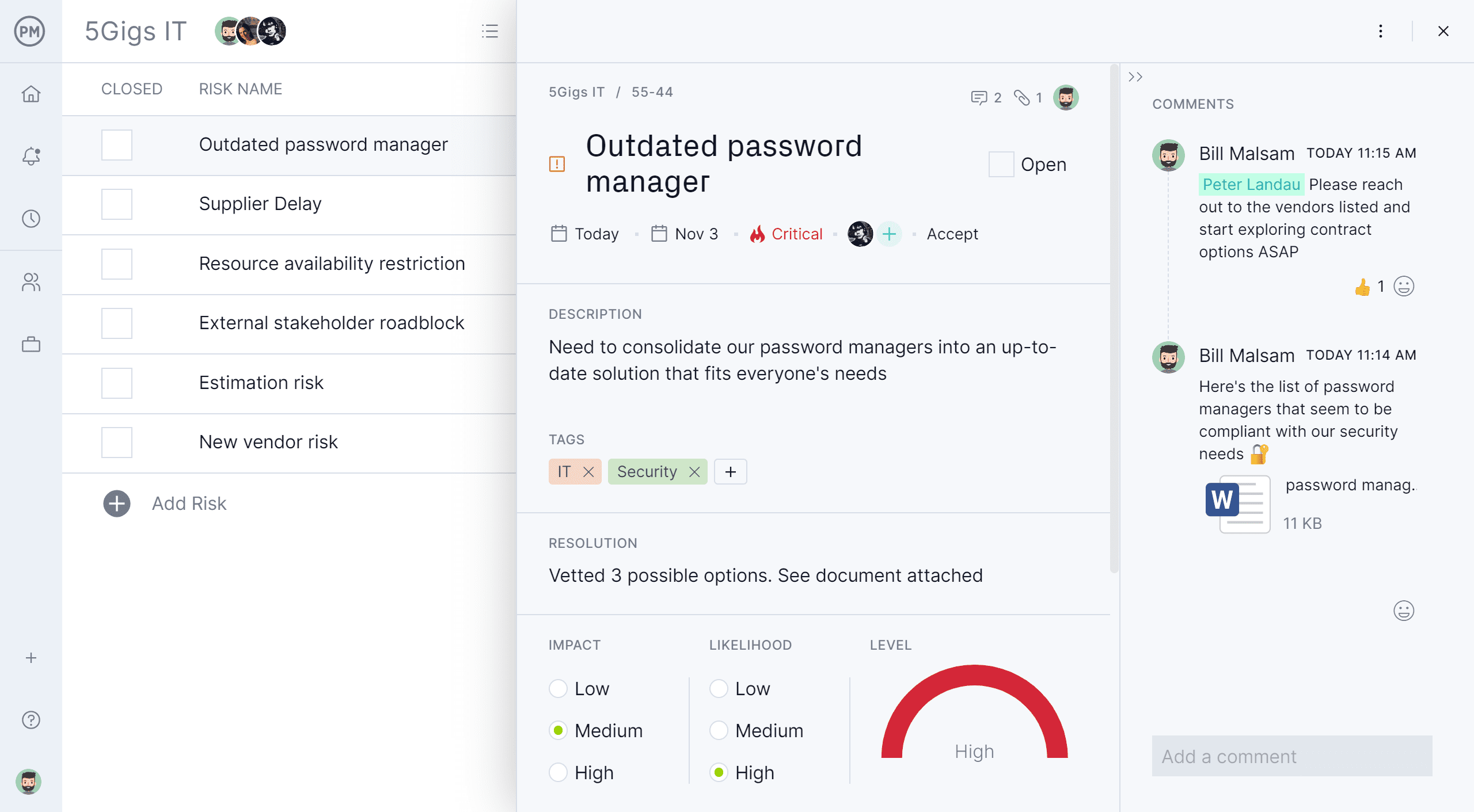This image showcases the interface of the 5 Gigs IT website. On the far left, there is a vertical menu bar that runs from the top to the bottom of the image. This menu includes several icons: a Home button, a Notification bell, a Clock icon, a Profile icon, and a Suitcase icon.

To the right of the vertical menu, we see a section titled "Closed and Risk Name". Under the "Closed" category, there are six checkboxes that can be marked, though currently, none are checked. The first risk listed under "Risk Name" is "Outdated Password Manager".

Further to the right, we see more details about the "Outdated Password Manager". This section includes a description area and a resolution section. Additionally, there are three selectable options for both the 'Impact' and 'Likelihood' of the risk.